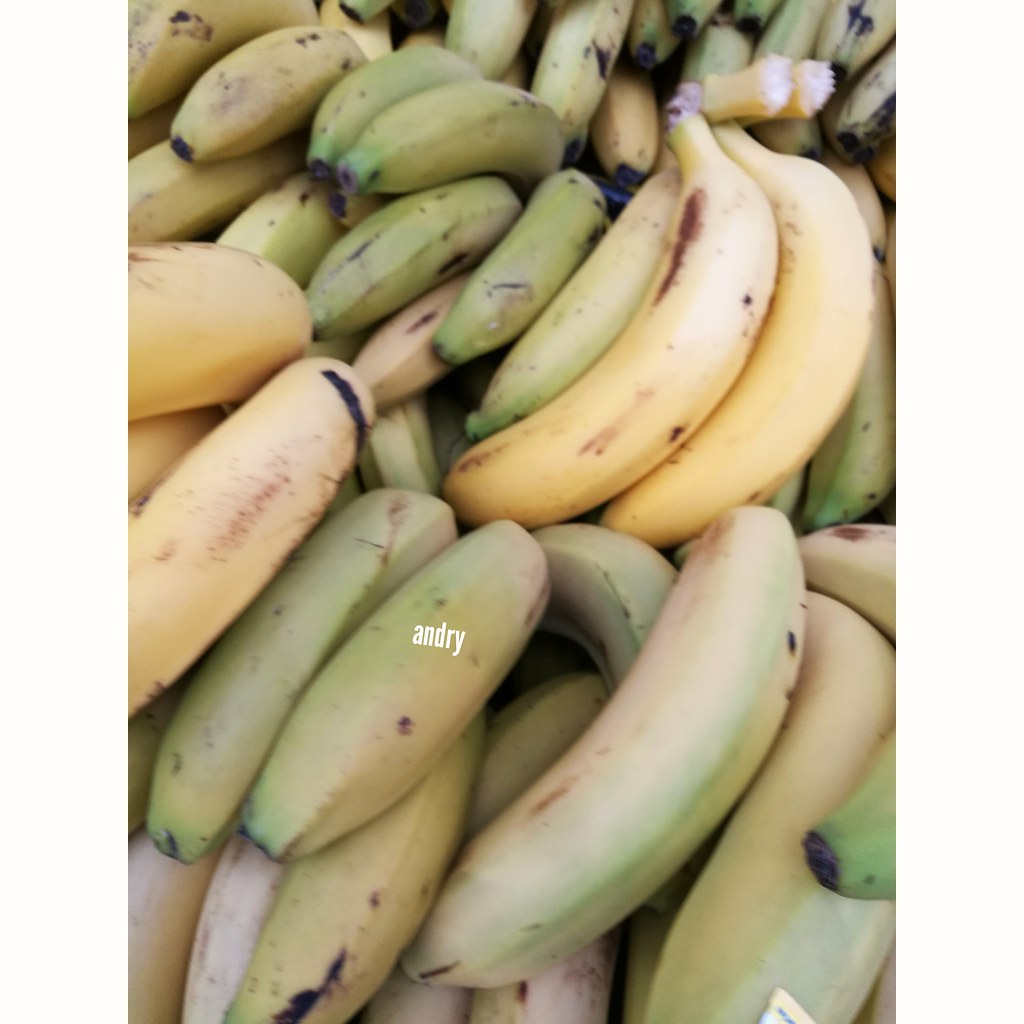The photograph captures an extensive close-up of various bunches of bananas, with a diversity in ripeness ranging from green to yellow, some showing a touch of overripeness marked by sporadic brown and black spots. Predominantly, you notice greener bananas, especially towards the left and bottom portions of the image, while the middle right area features primarily yellow bananas. Centrally located, about two-thirds down from the top, the word "andry" is prominently displayed in small, white lowercase letters. The majority of the bananas in the image have black spots. In the bottom right corner, a banana is adorned with a small, square sticker that is starting to peel off. The bananas, largely resembling the common Cavendish variety but with some appearing slightly larger, could hint at possible plantains among them.